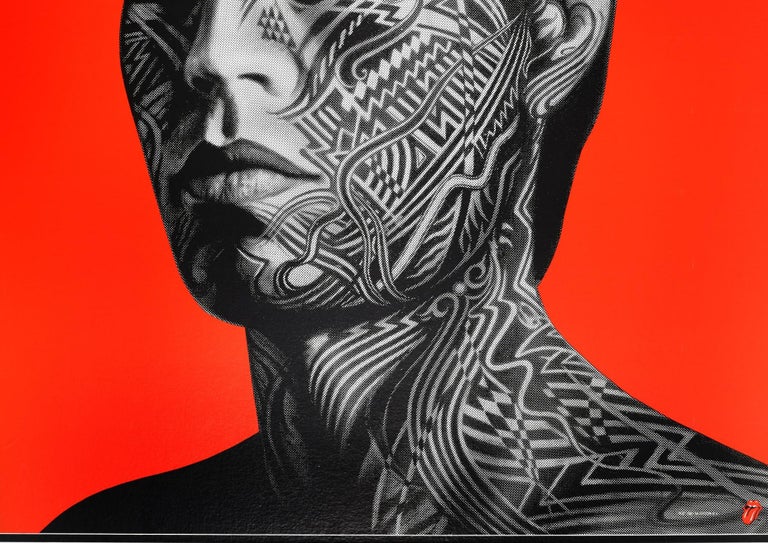This image appears to be graphic art with a bright red background. In the center, a person's upper body is depicted, focusing on the face, neck, and shoulders, but cropping out the eyes and top of the head. The individual is rendered in black and silver tones and is heavily tattooed with intricate geometric shapes and swirling lines that cover the majority of their face and neck, extending to the ears and top of the chest. Black hair is faintly visible. The left shoulder is in silhouette, adding a striking contrast. At the bottom right corner, there is the Rolling Stones logo featuring bright red lips and a protruding tongue. Beside the logo, there is small, unreadable text. The image is identified as an illustration of the album cover for the Rolling Stones' "Tattoo You," and it employs a heavy use of black and white on the subject against the vivid red backdrop.